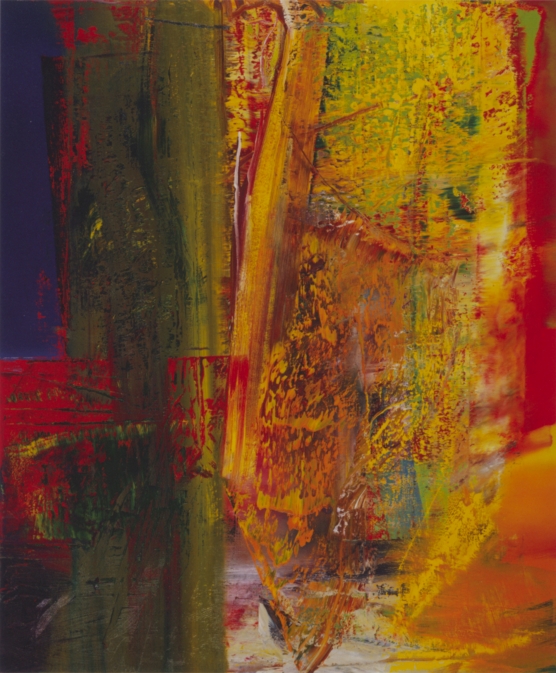This vertically aligned, rectangular image is an abstract painting awash with a vibrant array of colors. The painting features a thin strip of dark blue that runs from the middle to the upper left corner and a corresponding strip of dark red on the right side. Dominating the center is a vividly colorful blend, primarily featuring a splatter of yellow intermingled with touches of green, orange, and red. A narrow yellow strip runs vertically from the bottom to the top at the very middle.

In the left section, smoother lines blend yellow with green and transition to a predominantly brown area speckled with yellow spots. The right side showcases a strong presence of red and yellow hues. At the bottom of the painting, one can discern an outlined rectangular shape in red, overlaid with green and brown streaks. There's also a noticeable rounded yellow mark towards the bottom right, and a bit of white paint appearing subtly in the middle of the lower part of the image.

Overall, the painting is a complex interplay of splotches and streaks of color, portraying no recognizable objects but rather a chaotic yet harmonious fusion of colors working together in an abstract form.